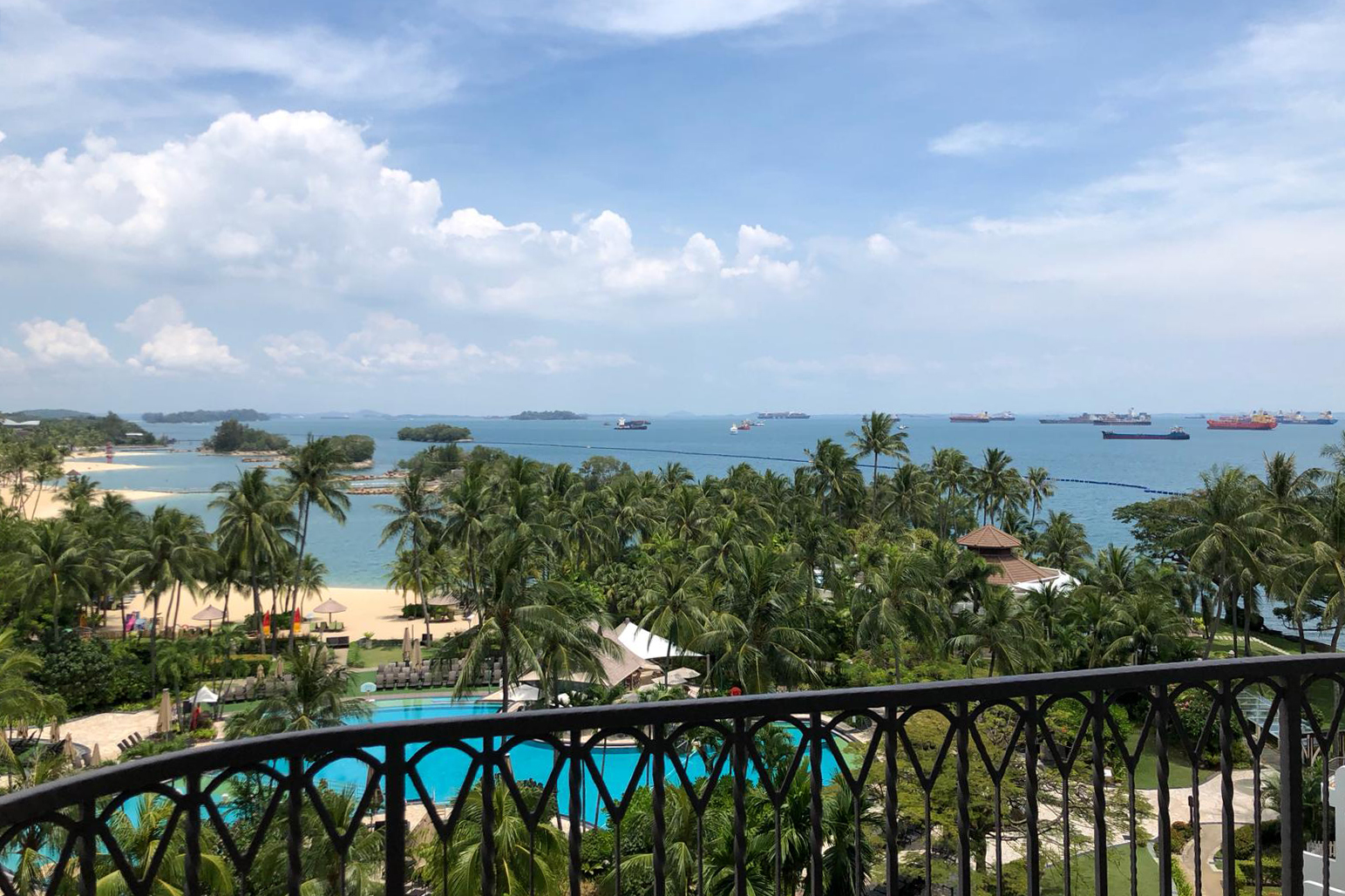This photograph, taken from a balcony with a black railing featuring a diamond-like decorative design between its spokes, captures a picturesque view of a tropical resort. The scene is dominated by tall palm trees, vibrant green patches of land, and winding walkways that lead to a large, in-ground pool with stunning light blue, almost electric blue water. The pool area is complemented by canopies and sandy spots that enhance the resort's allure. Beyond this, the ocean stretches into the distance, dotted with numerous large ships. The sky above is a mix of clear blue and fluffy white clouds, creating a tranquil yet dynamic atmosphere. An array of buildings, including one on the right with a brown chimney, are also visible, blending seamlessly with the scenic surroundings.